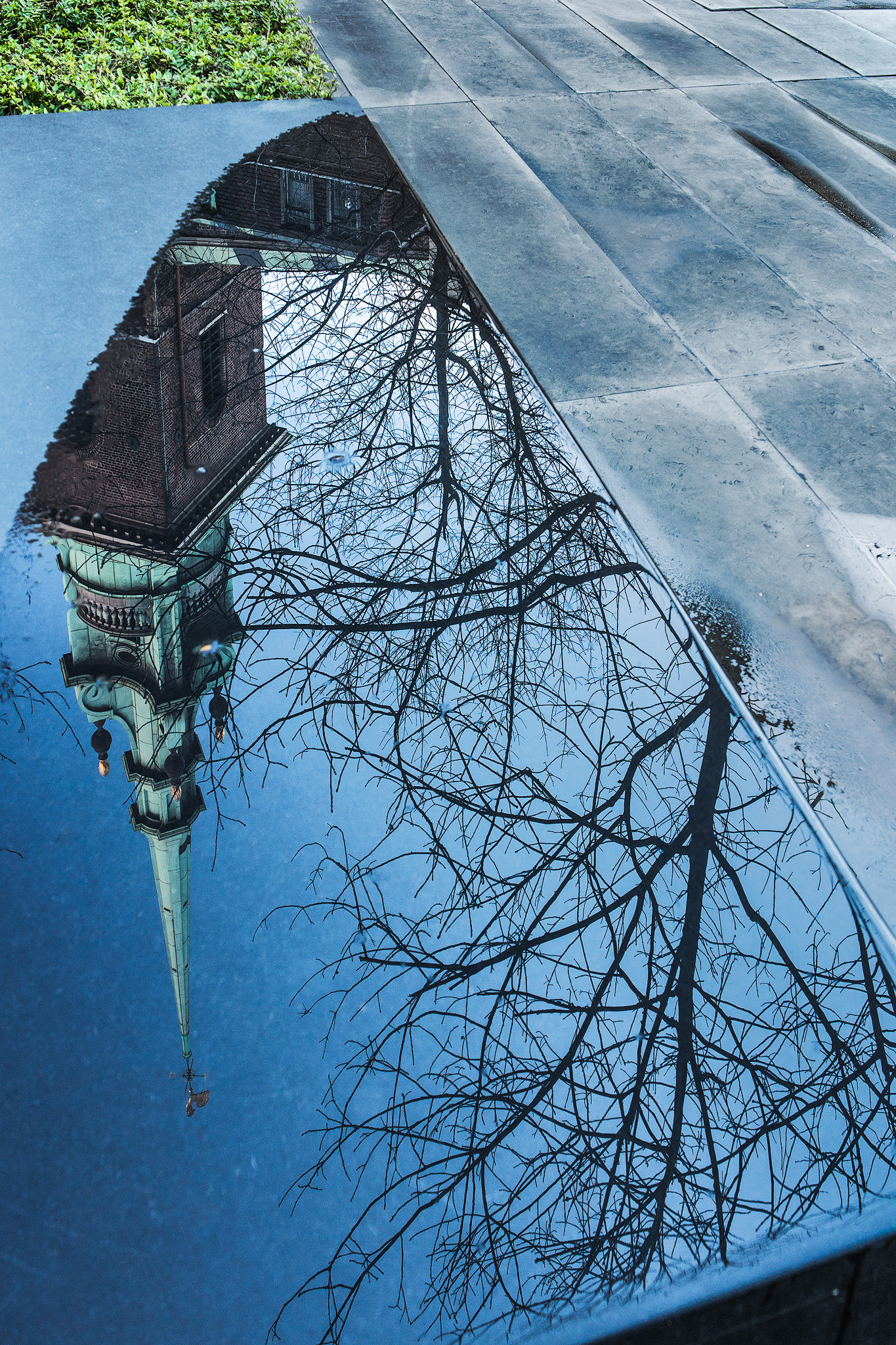This outdoor photograph captures the reflection of a building and leafless trees in a large, stagnant puddle on a wet sidewalk. The building, appearing inverted in the reflection, features a tall, narrow steeple with a worn blue-green, pointed top and a square, reddish-brown brick base reminiscent of a church or cathedral. Silhouettes of bare tree branches overlay the reflected blue sky and scattered clouds, adding depth and texture to the scene. On the right side of the image, adjacent to the puddle, lies a surface made of rectangular gray concrete pavers, suggesting a sidewalk or walking path. A small patch of green grass can be seen in the upper left corner of the photograph, captured in bright daylight. The overall color palette is dominated by shades of blue, gray, and green, with hints of brown and white.